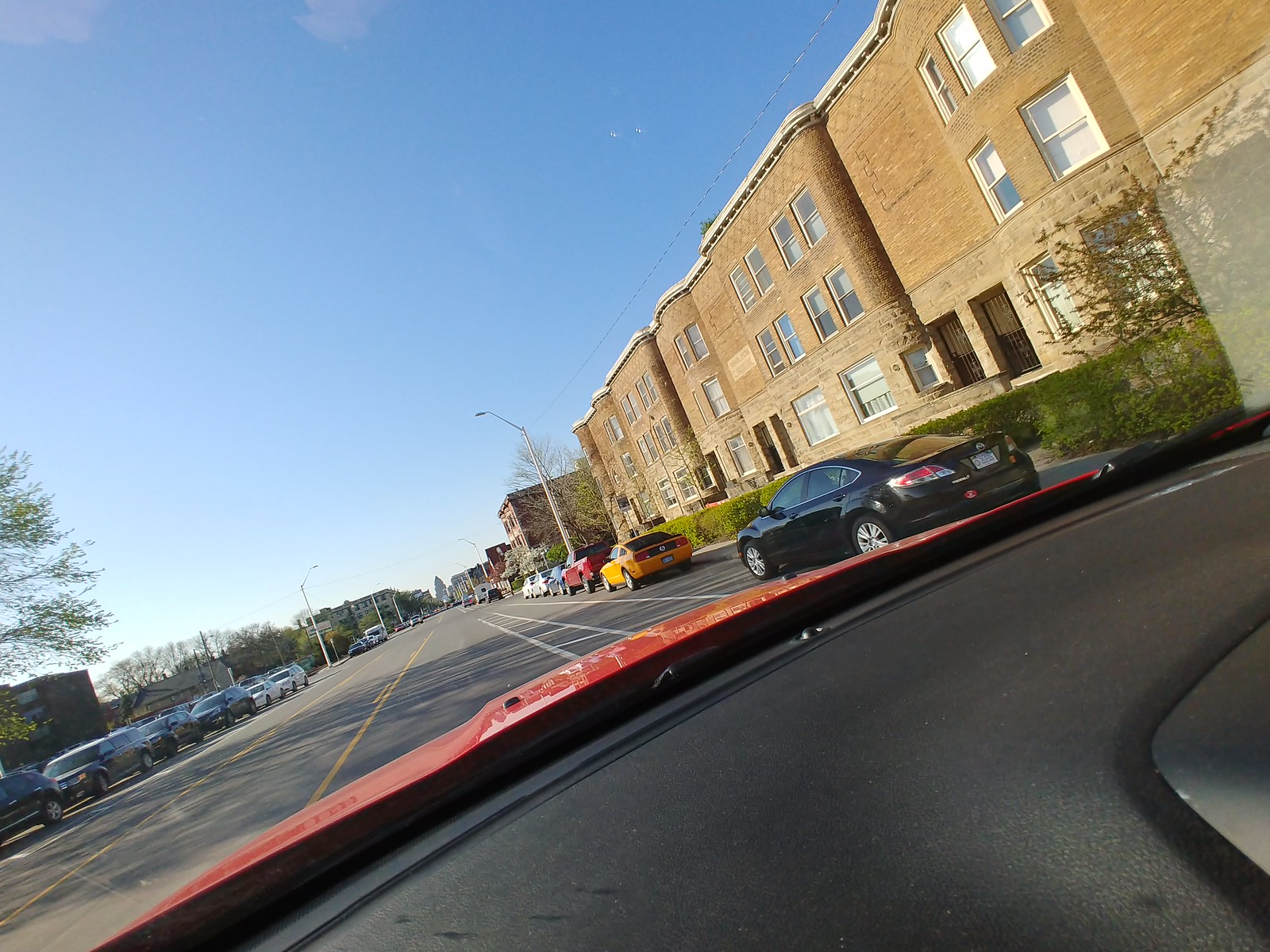This photograph captures an urban street scene viewed from the interior of a red car with a sleek black dashboard. The car is positioned on the right side of the road, which suggests the setting is likely in America. The street is lined with parked vehicles, including a clearly visible Nissan to the right, surrounded by other familiar American car models. 

On the right side of the frame, tan and brown stone and brick residential buildings dominate the scene. These three-story structures feature metal-barred doors and small front gardens with bushes, hinting at a neighborhood that values added security. The sky above is a vivid blue with scarcely a cloud in sight, indicating a clear, sunny day.

Notably, the photograph has a slight tilt to the right, causing the horizon to slant from the lower left to the upper right. In the background, a prominent conical or pyramid-shaped building rises, suggesting the skyline of a city or perhaps even the distinctive architecture of a state capital.

This detailed urban vista offers a snapshot of a quiet residential area under a bright sky, with a unique architectural landmark visible in the distance.